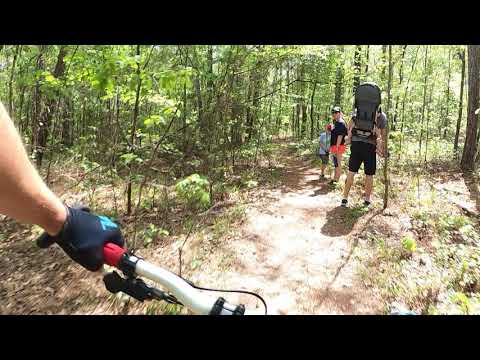In this image captured from the perspective of a cyclist on a narrow, rough forest trail, the scene is vibrant with greenery and surrounded by dense, tall trees. The cyclist, of Caucasian descent, has a gloved left hand on the handlebar, visible in the lower left corner. The cyclist's arm is bare, and you can see part of the handlebar. In front of the cyclist are three hikers. One hiker, with a large backpack and black shorts, is holding a walking stick in their right arm and is moving off the trail, seemingly to allow the cyclist to pass. Two other hikers, both wearing baseball caps and shorts, are standing to the side of the trail; they are talking to the hiker with the backpack and looking back towards the cyclist. The trail itself is brown dirt with patches of grass, and the wooded area is lush with green trees, creating a scene that speaks to the serenity of an outdoor adventure. The photograph also features a black footer and header but lacks borders on the sides, emphasizing the outdoor experience.